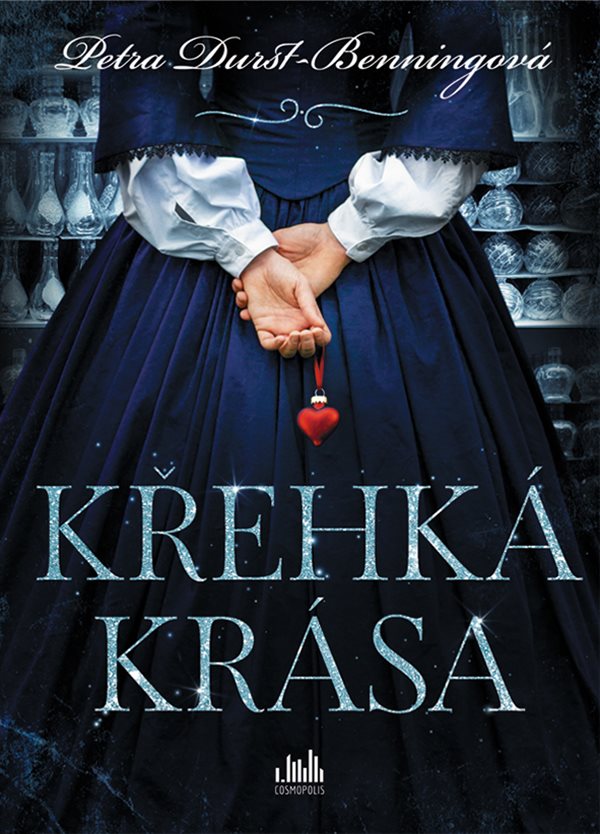The image, titled "Petra Darst Banning Gopher," appears to be a movie poster or magazine advertisement. It features the back of a woman, from the upper back down to almost her feet. She is dressed in a long, wide blue Victorian-style dress with many folds and a white shirt underneath, visible at the ends of her long sleeves. The woman, who has white skin, has her arms crossed behind her back and holds a red, heart-shaped pendant in her left hand. The text at the top, in cursive writing, reads "Petra Durst Beningova" with an accent mark, while the bottom third displays, in large all-caps sparkly letters, "K-R-E-H-K-A" with an accent followed by "K-R-A," also with an accent, and "S-A." The bottom center of the image says "Cosmopolis" in smaller text. In front of the woman, there are shelves filled with glass vases.